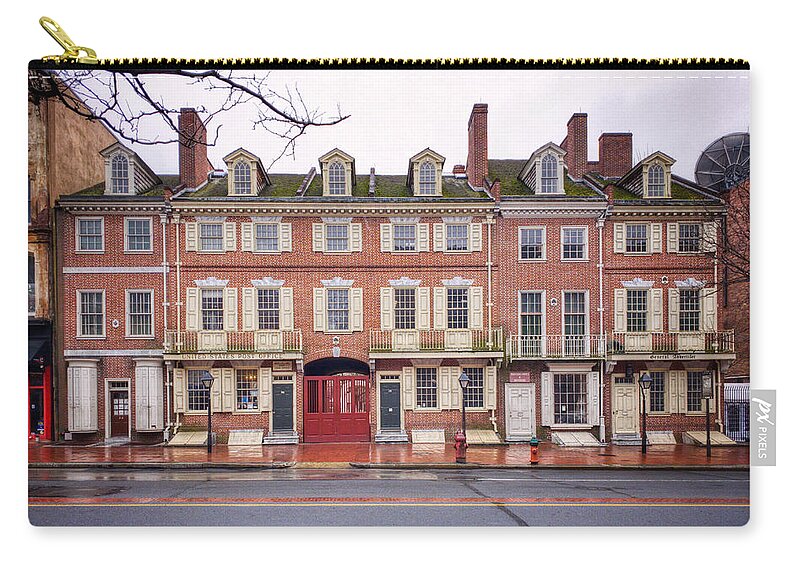This image shows a detailed photograph of a street scene printed on a zippered pouch. The gold zipper runs along the top edge with its pull tab positioned at the top left. At the bottom right, a small gray tag displays the company name, PX Pixels. The photograph, likely depicting a European cityscape, showcases a row of red brick buildings featuring multiple balconies, dormer windows, and chimneys. Dominating the scene is a striking red double door slightly to the left, suggesting access to a courtyard or similar area. The buildings are flanked by additional structures, one of which includes satellites. The view is straight-on, highlighting three distinctive floors plus an attic. Various white and yellow windows punctuate the façade. In the foreground, there are fire hydrants, light poles, and cellar access points along the sidewalk. The street below, marked with red and yellow stripes, appears wet, indicating a rainy day. Sparse branches hang in from the top left corner, devoid of leaves, reinforcing the rainy and perhaps overcast atmosphere.